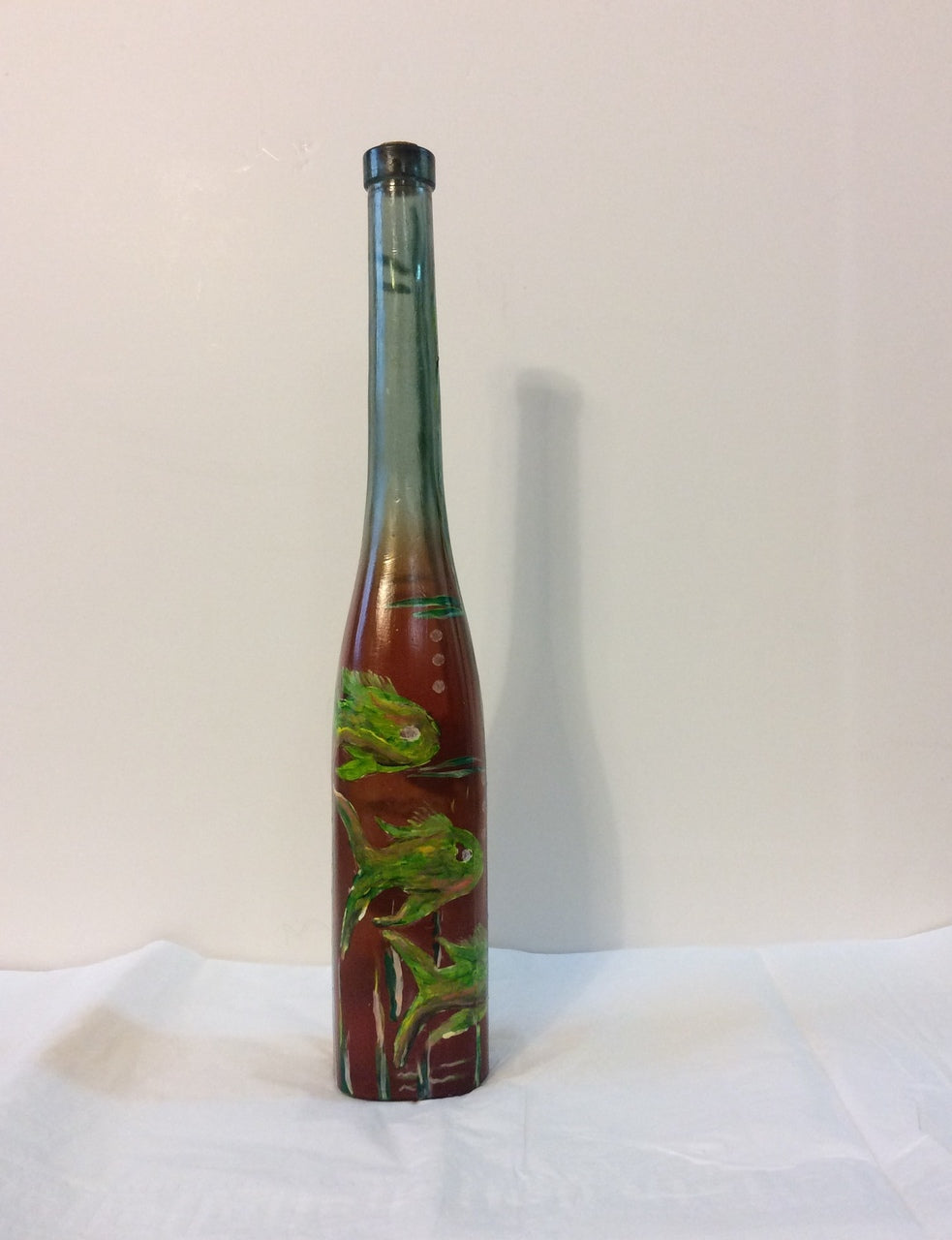In this image, a tall, narrow green bottle with a long neck and a black cap stands prominently at the center. It rests on a piece of slightly wrinkled white fabric, which adds texture to the scene. The background is a beige-colored wall that highlights the bottle's details. The bottle has a distinctive design featuring a red and green pattern that starts below the neck and extends to the bottom. This intricate pattern depicts green fish with red and white eyes, swimming in what appears to be red water. The fish are detailed with small streaks and bubbles. Subtle shadows of the bottle can be seen both on the fabric and the wall, adding depth to the composition. The overall detail makes it unclear what liquid, if any, is within, as the bottom part of the bottle remains opaque and mysterious.